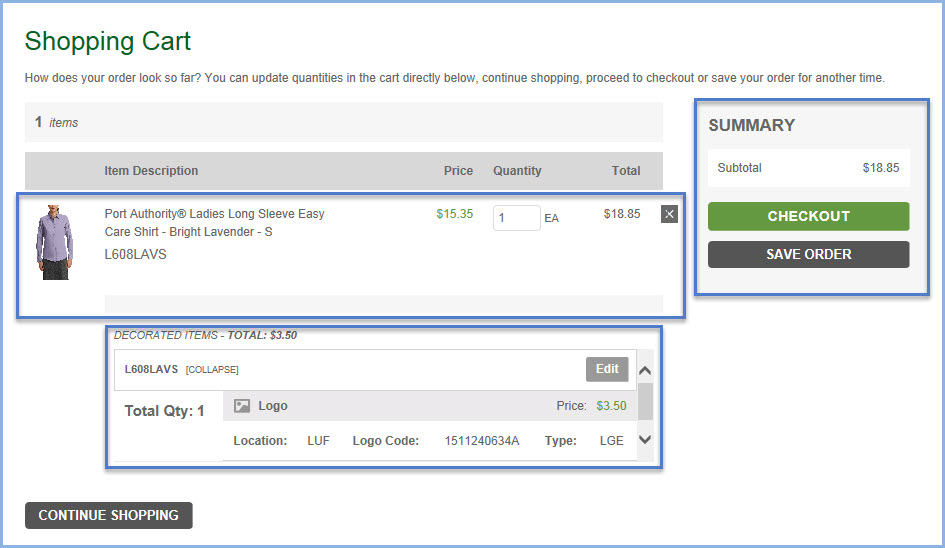The screenshot features an online shopping cart interface with a clean white background bordered in blue. In the upper left corner, green text reads "Shopping Cart," alongside the message, "How does your order look so far? You can update quantities in the cart directly below. After shopping, proceed to checkout or save your order for another time." 

Directly below this is the cart summary against a gray background, which includes columns for "Item Description," "Price," "Quantity," and "Total." Listed is the "Port Authority Ladies Long Sleeve Easy Care Shirt" in Bright Lavender, size Small (product code L608LAVS), priced at $15.35. The quantity is set to 1, bringing the total to $18.85.

Additionally, a section is dedicated to "Decorated Items," priced at $3.50 each. This product customization includes a logo with the code 1511240634A, placed at the location denoted as "LUF," in a large size.